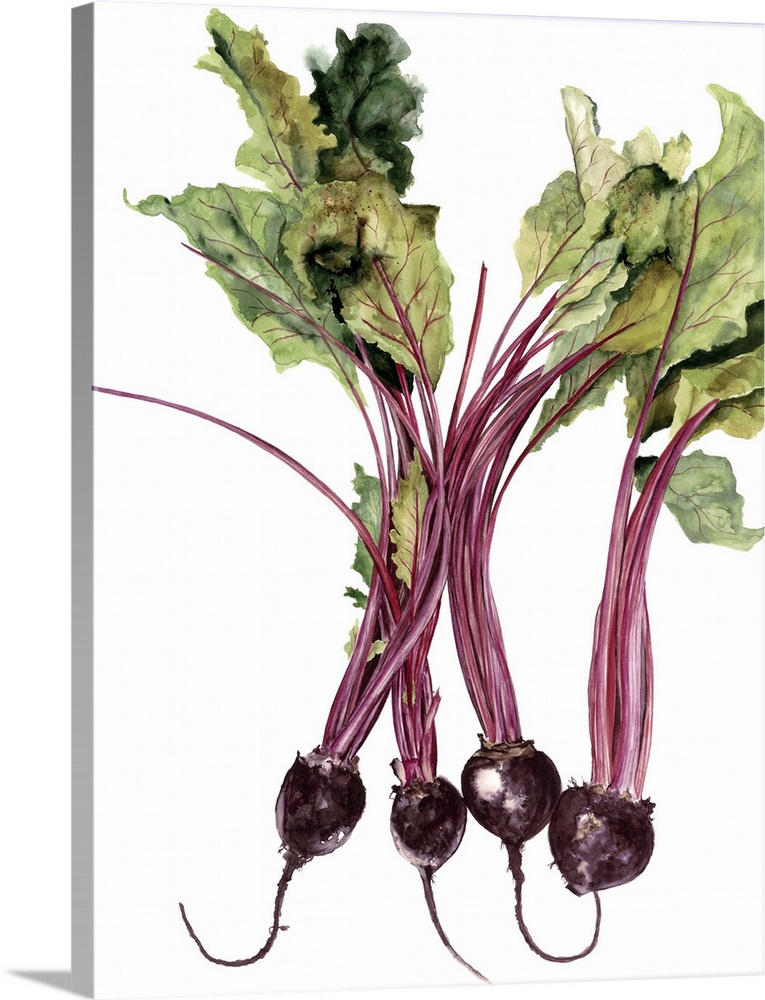This is a photorealistic watercolor painting of beets on a white background. The composition features four intact beetroots with their roots, stems, and leaves still attached. The beetroots are a deep purplish-red hue, and their roots curl into hook shapes, adorned with fine root hairs. The stems are a lighter reddish color and lead up to the leaves, which vary from a dark forest green to a lighter yellow-green, with reddish-purple veins prominently running through them. The vibrant colors and intricate details of the leaves and roots highlight the hand-painted watercolor technique, giving the beets a lifelike and dynamic appearance.